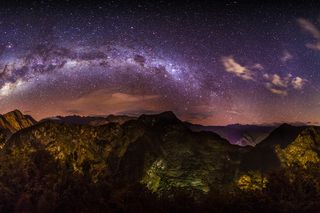A dark and serene night scene captures the viewer’s attention with a mesmerizing mix of artistry and natural beauty. Featuring a rugged foreground of indistinct, dark hills or mountainous forms, the real spectacle lies in the sky above. A stunning celestial backdrop painted in hues of purple, black, gray, and tinges of tan and pink spans the horizon, evoking the grandeur of a galaxy. Whisps of clouds interlace with the vast expanse, adding depth and complexity to the scene. Despite the overall darkness, the intricate details of the sky contrast notably with the shadowy silhouettes of the mountains below, making the scene feel both tranquil and otherworldly. The precise medium—be it a high-definition photograph or a digital painting—remains ambiguous, yet it unmistakably conveys a sense of peaceful contemplation, inviting viewers to lose themselves in the infinite.